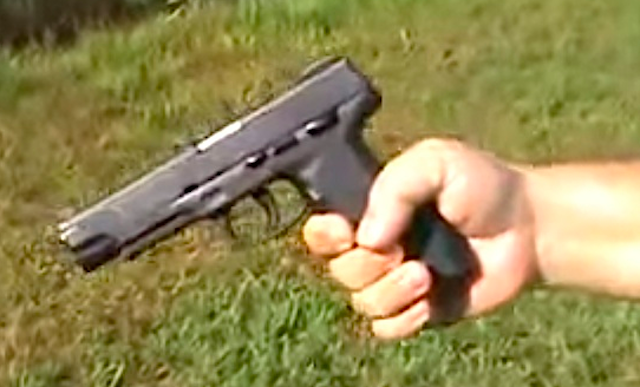The image depicts a blurry, grainy scene of a white, somewhat plump hand gripping a small, plain black handgun. The gun is being held with fingers wrapped around the handle, and the finger distinctly rests below the trigger, indicating it is not in a firing position. The gun is angled downward towards the bottom left side of the frame. The background shows an indistinct grassy area, suggesting an outdoor setting. Despite the low image quality, it's clear that the fingernails are clean and unpainted, and no advanced modifications like a silencer are present on the compact, all-black gun.